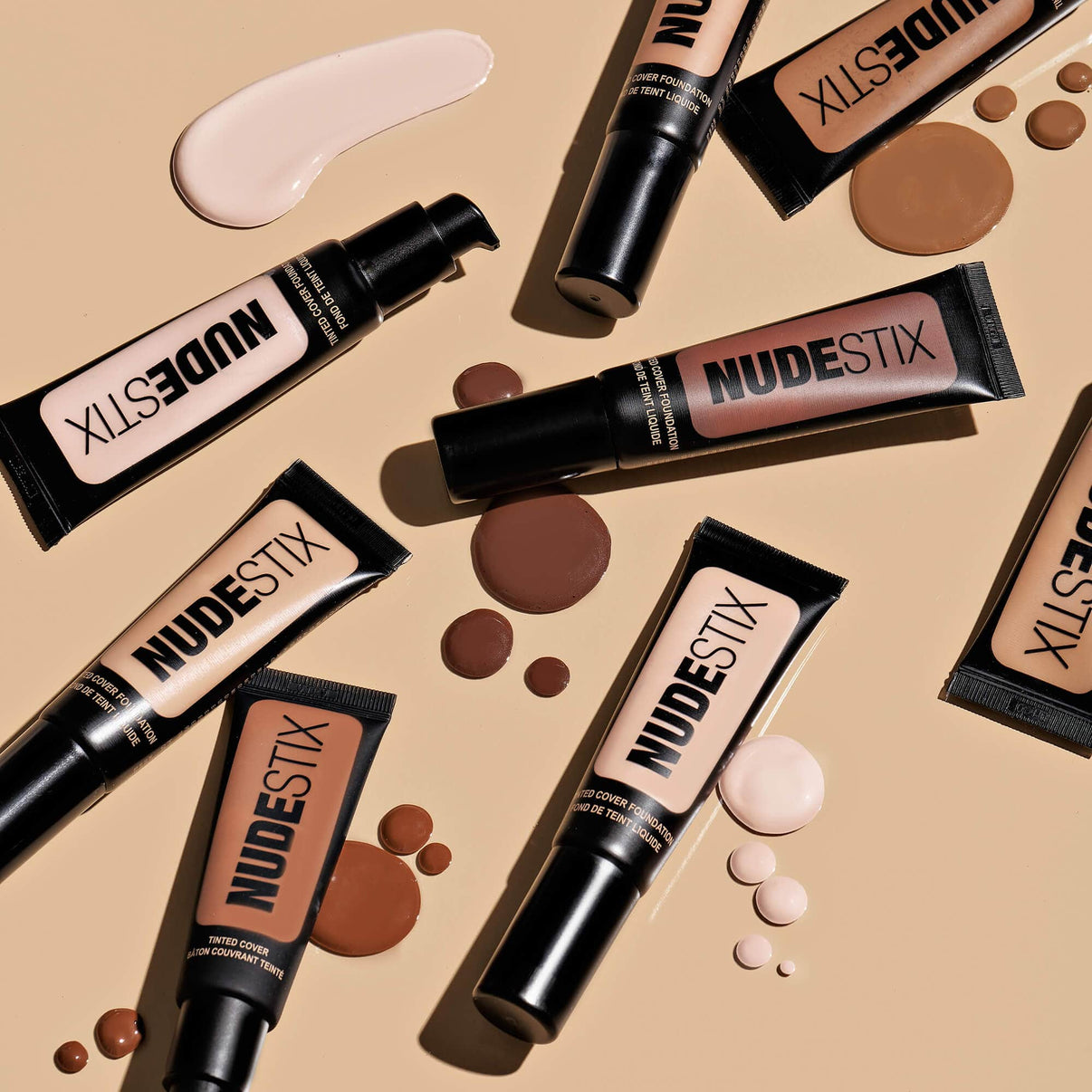The image showcases an assortment of NUDESTIX makeup products spread out on a dark tan background. There are seven or eight small containers prominently labeled "NUDESTIX" in black font, set against varied shaded backgrounds including dark brown, peach, and pinkish white. These containers illustrate a diverse range of skin tones, from pale to dark, representing different shades of cover foundation. Surrounding these products are multiple blobs of liquid foundation matching the closest container’s shade, enhancing the visual display of the color spectrum. The NUDESTIX tubes and their associated drops are carefully placed, projecting a well-organized yet aesthetically pleasing presentation of the product line. Some containers are partly cropped out, emphasizing the variety and abundance of available shades.